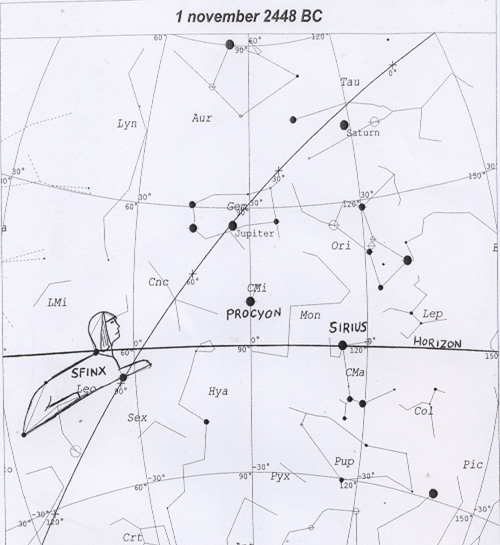This detailed sky map, titled "1 November 2448 BC," appears to be an ancient astrological chart drawn on a faded page with black ink. The map features a grid of curved horizontal and vertical lines with markings indicating different degrees at their intersections. Across the chart, various celestial objects and constellations are meticulously labeled, including Sirius, Procyon, and abbreviations for Orion's Belt. A horizontal line labeled "Horizon" runs about a third of the way up the map, intersecting with a diagonal, slightly arcing line extending from the bottom left to the top right. This diagonal line has dots along it, likely representing stars. Notably, a prominent line drawing of the Sphinx is positioned diagonally near the intersection of these lines. The map includes additional three-letter constellation abbreviations such as LYN, AUR, TAU, and LNI, enhancing its detailed portrayal of the night sky.